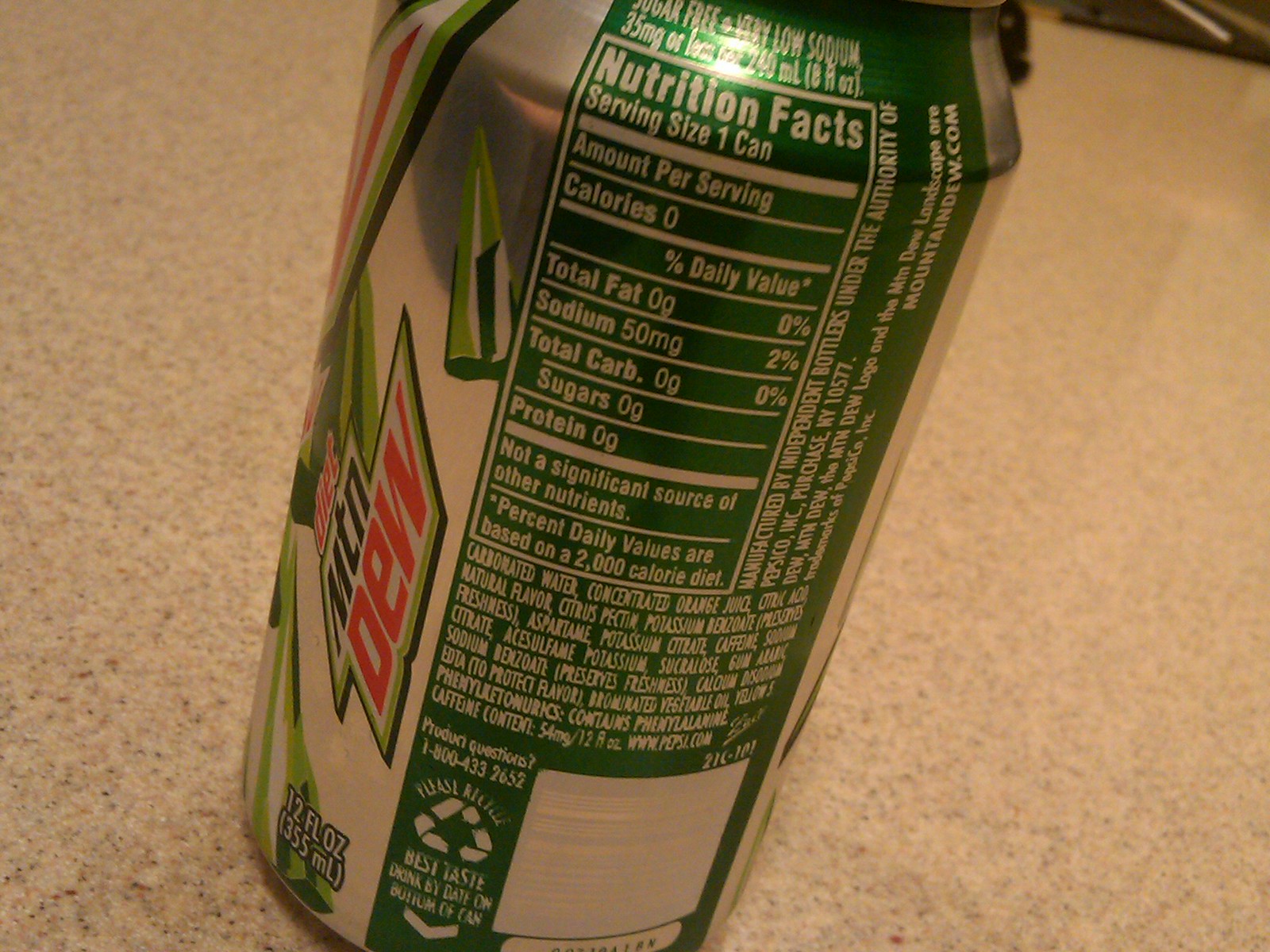The photograph showcases a can of Diet Mountain Dew placed at a slight angle on a matte beige granite-style countertop. The can features the recent Mountain Dew logo, suggesting it is a fairly recent product. It exhibits the characteristic red, green, and silver color scheme. The focal point of the image is the detailed nutrition label, which is fully visible and includes information such as "Serving Size 1 can," "Calories 0," and "Sodium 50 mg." The label also notes "Total Fat 0," "Total Carb 0," "Sugar 0," and "Protein 0," with a reminder that Percent Daily Values are based on a 2000 calorie diet. To the left side of the can, parts of the Mountain Dew logo and the liquid quantity are visible. Additionally, the list of ingredients and a recycling symbol are present. In the upper part of the can, glare from a light source is noticeable. A dark object with some white and beige parts is partially visible in the upper right corner, slightly cut out of frame. Overall, the can appears quite shiny and metallic.